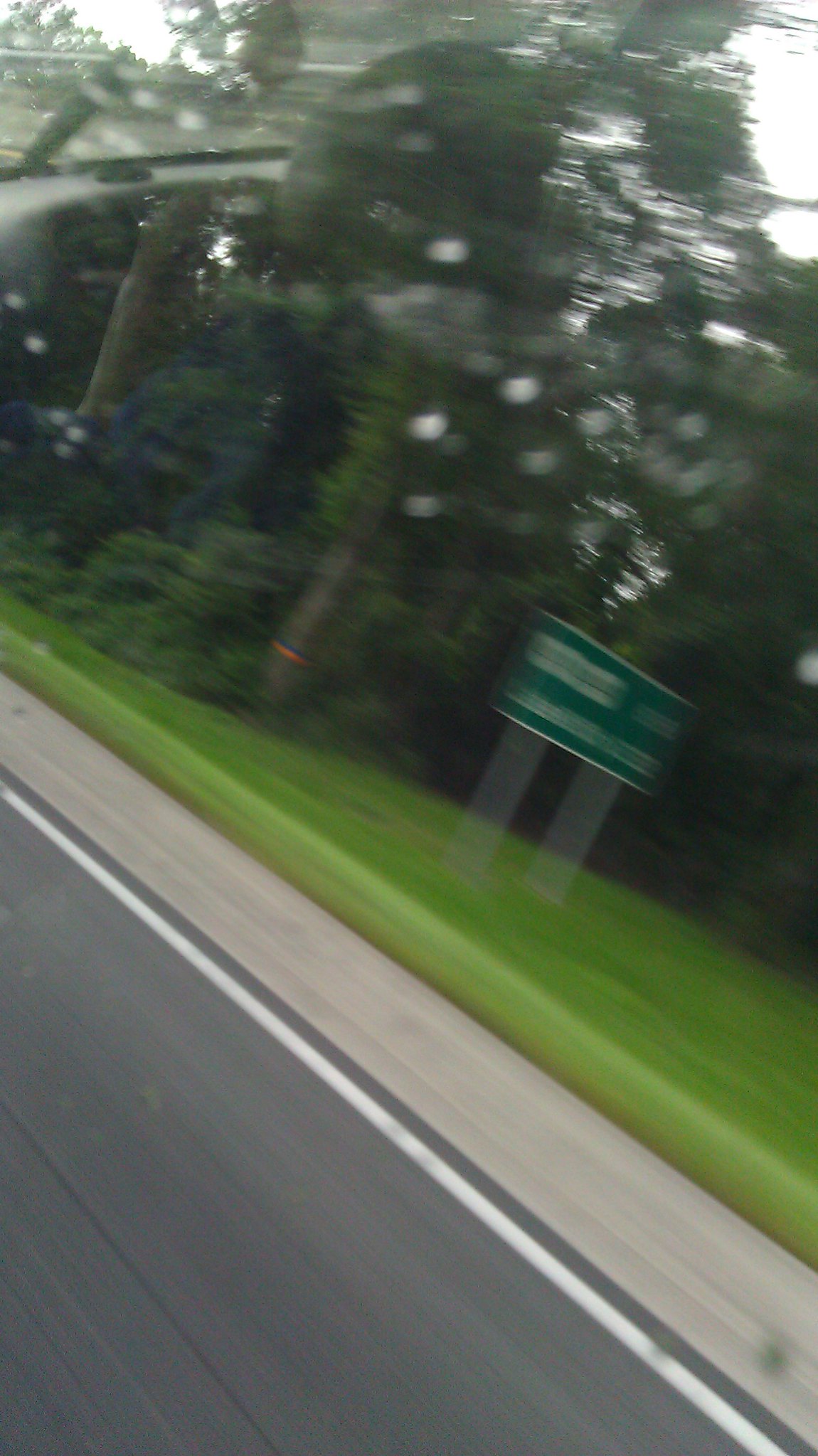Captured from a moving car on the highway, this image portrays the dynamic blur of rapid travel. At the center, a small green highway sign is almost unreadable due to the motion blur, indicating a swift passage. The sign is modest in size and situated not too far from the ground, surrounded by an overgrowth of tall trees and dense brush. Below, a strip of meticulously manicured, vibrant green grass contrasts sharply with the wild foliage above. The edge of this grassy strip appears unusually curved and smooth, almost giving off an artificial, plastic-like impression. The photograph also captures the clear shoulder of the road with a distinct white line marking its boundary, reinforcing the scene's highway setting.